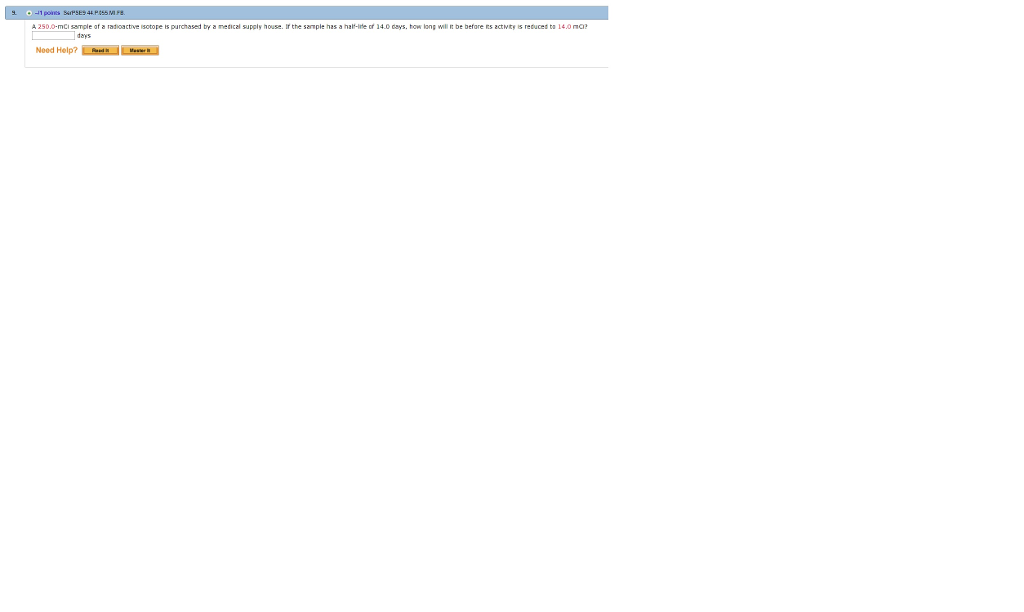The image features an assortment of elements laid out in a detailed manner. 

In the top-left corner, there is a prominent blue rectangle. Inside this rectangle, the letter 'B' can be found. Accompanying this is a red text "250" which appears bold and distinct against the blue backdrop.

The primary content of the image seems to be a scientific problem regarding a radioactive isotope. Specifically, it mentions a 250 mCL sample of a radioactive isotope purchased by a medical supply house. It states that the isotope has a half-life of 14 days, and the task is to determine the duration required for the activity of the sample to reduce to 14 mCL.

There is also a mention of various locations and calls for assistance, including a reference to Orange Texas with a note saying "need help" followed by "Read it." 

The entire content is set against a white background, making the text elements more noticeable despite their grainy appearance. The visual clarity is reduced, with the text described as "very grainy, not much visible," which suggests that the image quality may be low.

This detailed mishmash of elements invites viewers to engage with a complex scientific query amidst scattered callouts and encoded messages.